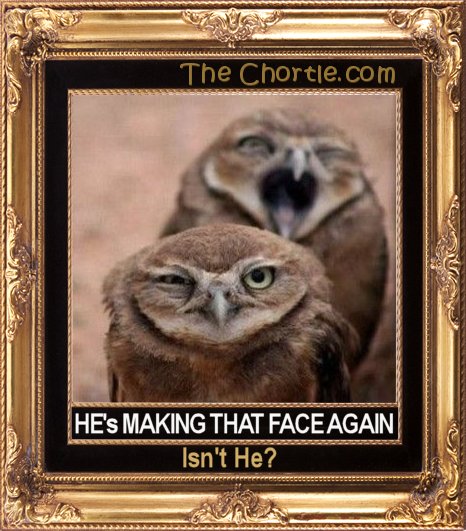The image depicts a poorly edited digital meme featuring two owls with distinct expressions. The foreground owl is winking, while the background owl has its beak wide open in what appears to be a grumpy or goofy expression. The overall quality of the image is low, with a blurry beige background and an ornate, shiny gold gilded frame adorned with intricate embellishments. Light reflects off the frame, emphasizing its opulence in contrast to the meme's crudeness. Text is present on both the upper and lower parts of the image; the top reads "TheChortle.com," while the bottom, on a black matte with white font, states, "He's making that face again, isn't he?" No additional objects or figures are present, and the context of the meme remains unclear aside from the reference to TheChortle.com.